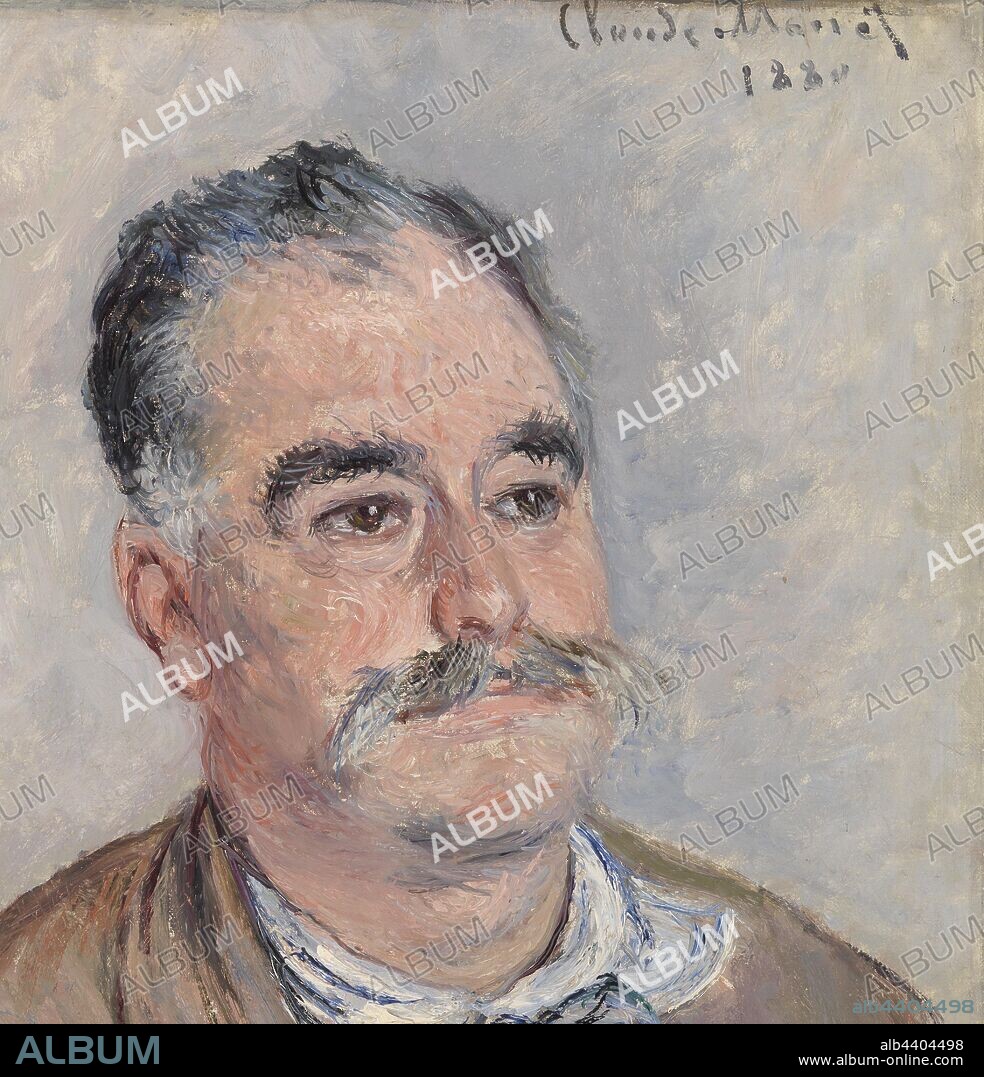This image showcases an artist's rendition of an elderly white man, seen from head to shoulders, painted with rough, exaggerated brushstrokes that suggest it could be an oil or acrylic painting. The man has thinning black and gray hair, with gray roots and darker sides, alongside shaggy eyebrows. His facial features include large brown eyes and a noticeable handlebar mustache that extends past his lips, primarily gray with touches of black in the middle. He is depicted wearing a brown shirt with a white undershirt peeking through the collar and is gazing slightly off-center towards the right, with his chin subtly raised. There is a black bar at the bottom of the image, where the words "ALB4404498" and "www.album-online.com" are displayed in light gray text. Additionally, the word "album" appears as a watermark in light gray or white, diagonally repeating across the entire image, contributing a faint, almost transparent overlay. This detailed portrait gives a vivid impression of the gentleman’s character and the artistic techniques used to create this striking image.